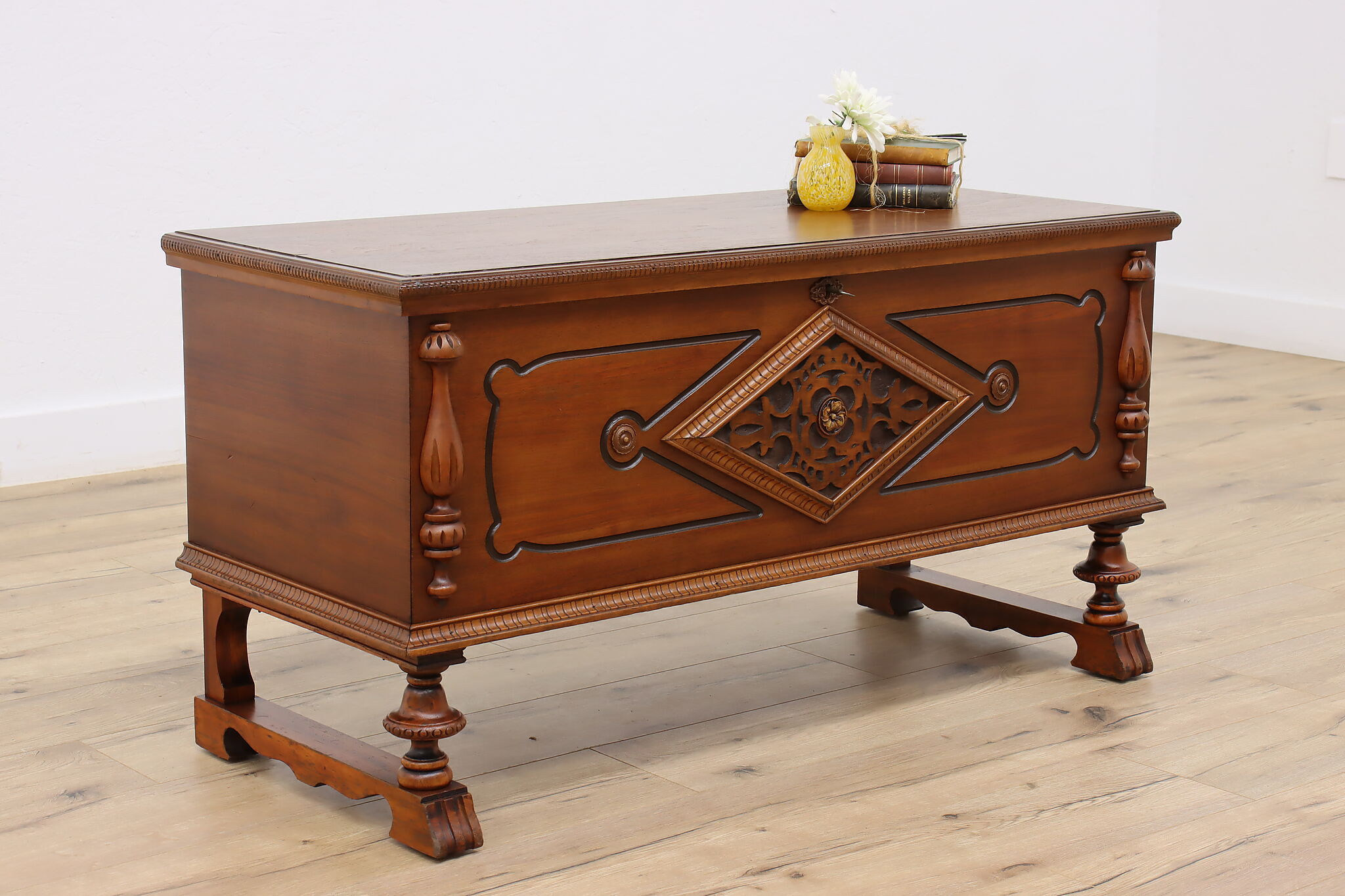This image showcases an ornate chest that can double as a coffee table. The chest is made of a golden medium brown wood, possibly walnut, adorned with intricate carvings and moldings. Its flat top features a keyhole with a key inserted, and it supports a yellow vase with wilting white flowers alongside a stack of three tied books. The front of the chest is heavily decorated, displaying a diamond-shaped centerpiece with a Celtic-inspired floral design. The chest is supported by four legs; the front pair are rounded and lathed with spherical details, while the back legs are straight with concave curves, all resting on carved wooden pedestals. The surrounding room features a light-colored wall and a hardwood floor, highlighting the chest's elegant and functional design.